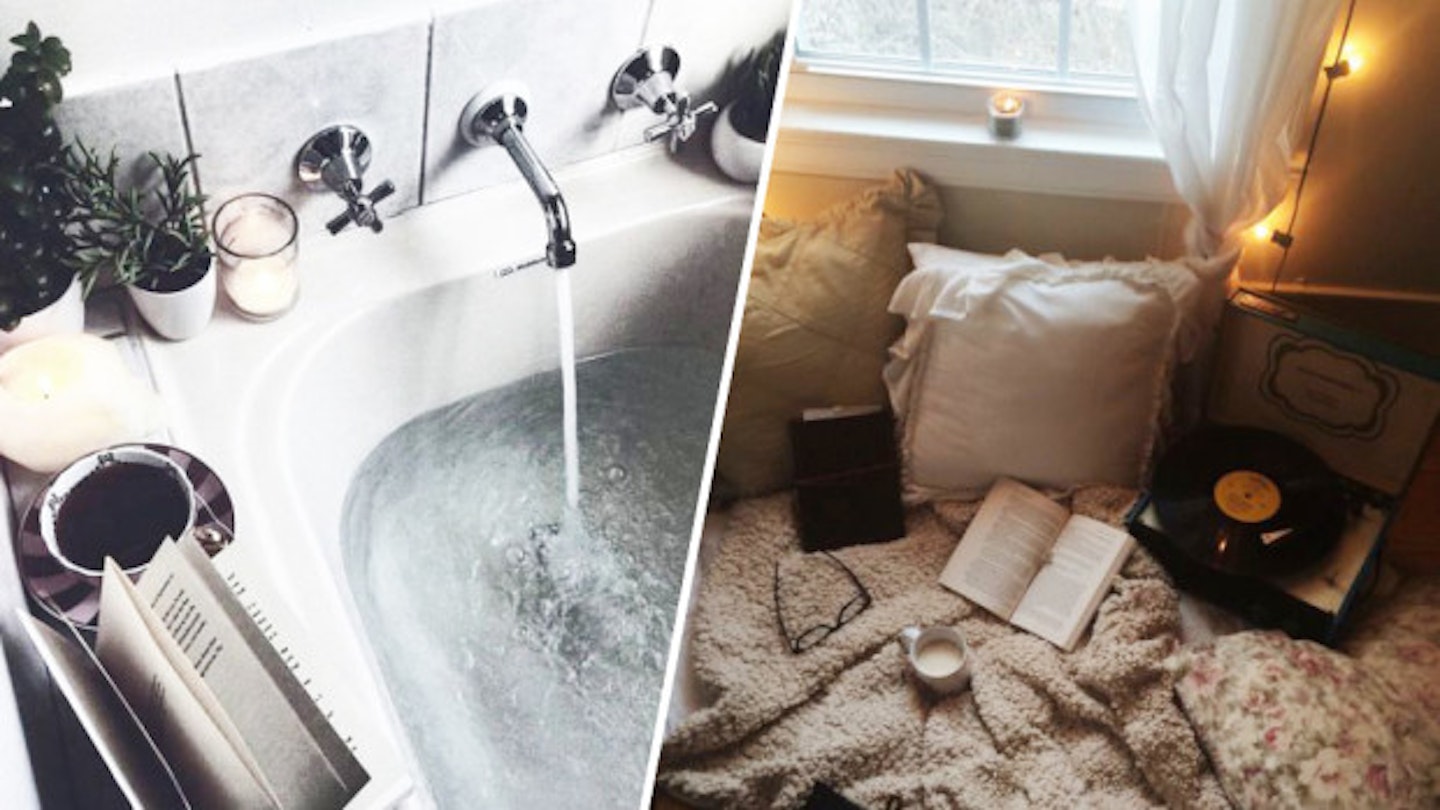The image is an indoor collage comprised of two photographs separated by a white line running diagonally through the center. The left photograph is monochromatic and features a serene bathroom scene with a white bathtub being filled with water from a stainless steel faucet. Around the bathtub, there are small, white potted plants and a glass jar candle, enhancing the relaxing atmosphere. A book and a cup of dark liquid rest on the bathtub's edge, perfect for a cozy reading session.

The right photograph captures a cozy nook beside a window adorned with white curtains and twinkling yellow lights. The scene includes a beige blanket spread on the floor, with matching beige and white pillows propped against the wall. An open book and a pair of eyeglasses lie next to a cup of milk, inviting relaxation. Additional elements like a record player and a flower-print blanket add to the sense of comfort and leisure.